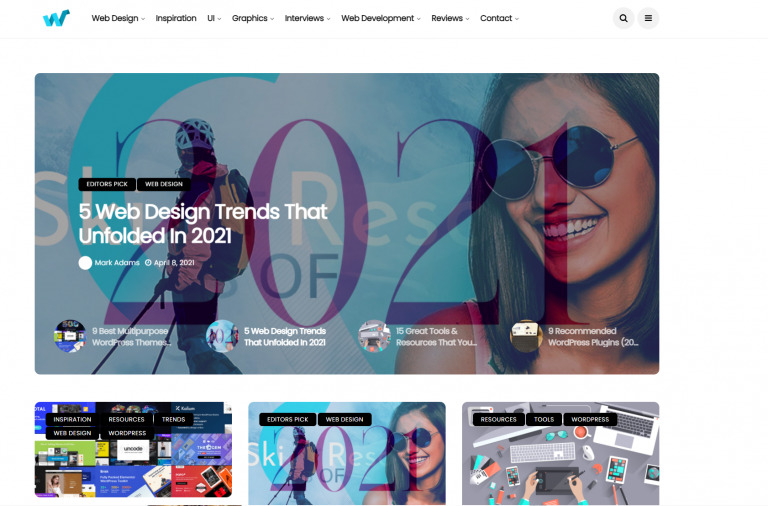The image depicts a series of computer screen graphics from a website. At the top, a navigation bar features icons, including a possible Microsoft icon, a magnifying glass for zooming, and a distinctive "W" logo resembling a stock market graph. The menu items read: Web Design Inspiration, Graphics, Interviews, Web Development, Reviews, and Contact, indicating it's a web design or tech-related company.

Dominating the display is a large central rectangle featuring a photograph of a smiling young woman with straight brown hair just past her shoulders, donning a sleeveless top and mirrored sunglasses. To her left is a smaller image of an individual with ski poles, a backpack, and a helmet, suggesting trekking or mountain climbing. Overlaid on these images is the bold white text "Five web design trends that unfolded in 2021," with "2021" prominently displayed in purple. Background letters in white are faintly visible.

Below this primary image are three smaller rectangles. The center rectangle is a smaller replica of the main image. The right rectangle shows an overhead view of a desk, complete with keyboards, thumb drives, phones, a coffee cup, and a tablet, and features black boxes with white text: Resources, Tools, and WordPress. The left rectangle presents a montage of illustrations, possibly related to designing, with accompanying menu items.

Additionally, circular thumbnail images at the bottom highlight various topics: "9 recommended WordPress plugins," "15 great tools and resources that you [Unfinished]," and "5 web design trends that unfolded in 2020-21."